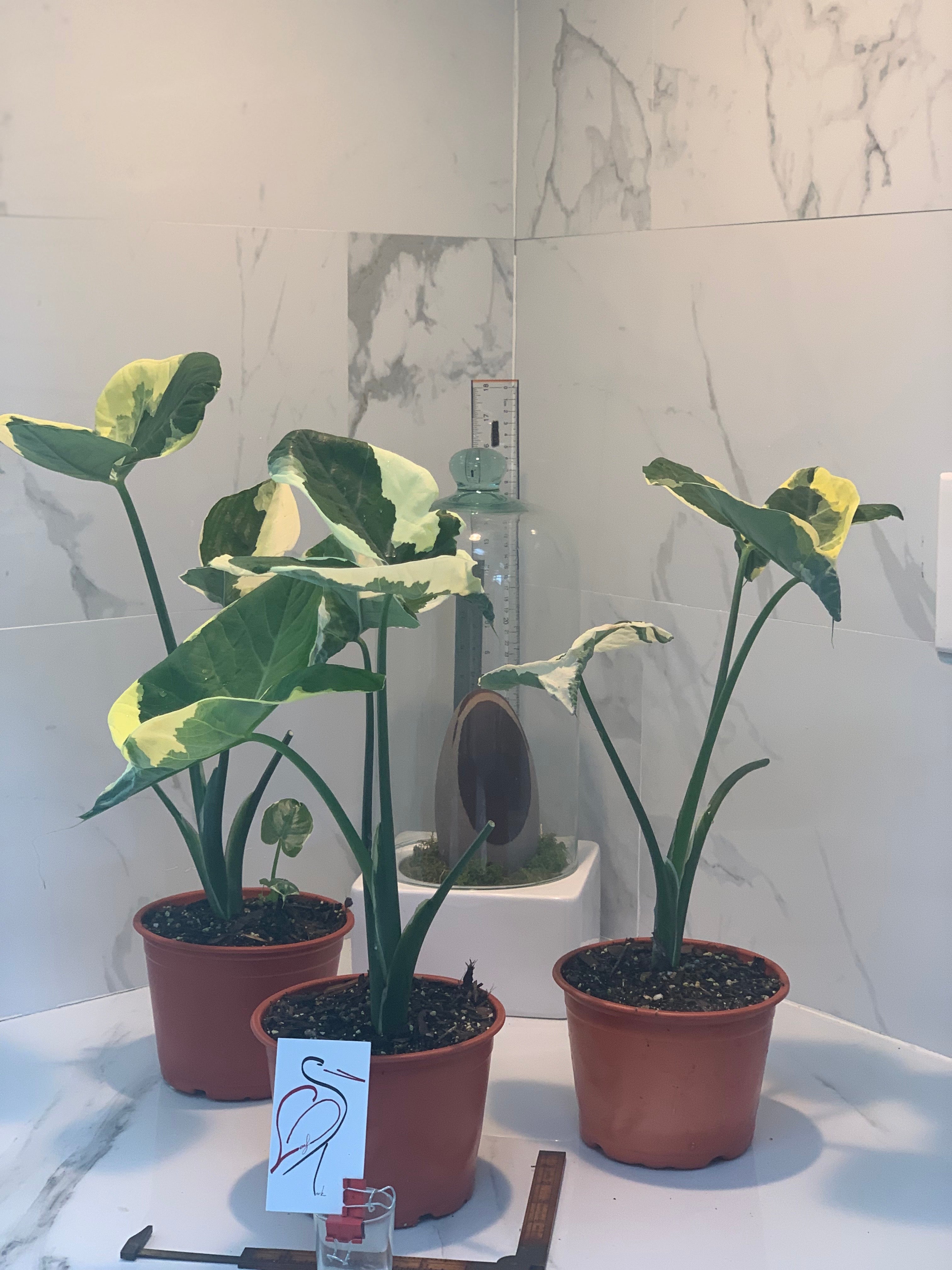The image features three tall plants with variegated dark green and cream-colored leaves, growing in plastic terracotta-colored pots on a white and gray Carrara marble countertop. The wall behind them is tiled with matching white and gray Carrara marble. A white card with a stylized red sketch of a pelican is placed in front of one of the pots. In the back corner, a tall, clear cloche-style lid on a white base covers an object, possibly a statue, accompanied by a ruler leaning against the wall. The plants also bear yellow flowers among the leaves. The setting creates a clean and elegant appearance, highlighting the lush greenery of the plants against the polished marble background.